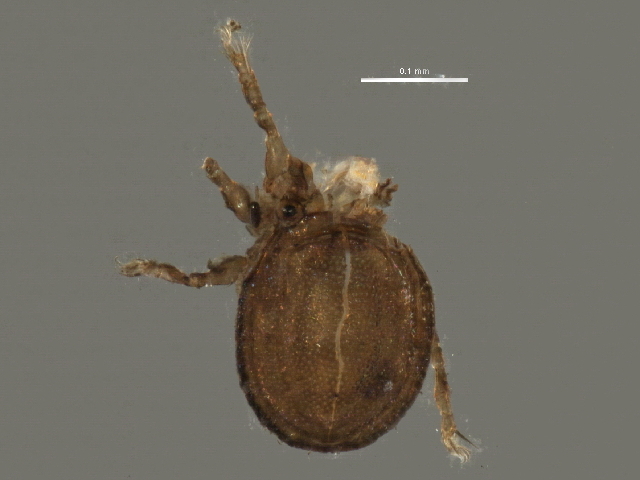This image shows a close-up, microscopic view of a small insect or mite with a distinctive appearance, set against a dark gray background. The image includes a horizontal white bar labeled "0.1 mm" above the insect, indicating the scale of magnification. The insect's body is an oval shape with a turtle-like shell characterized by a central crack and numerous tiny circular structures around it, possibly representing fine hairs. The shell displays varying shades of green, with the central crack being a lighter green against a darker green shell. The insect appears to have multiple legs: one leg extending upwards, another leg pointing to the left, and one leg pointing downward. Additionally, a fuzz-like, thread-like white substance is visible near the top of its head. The insect has beady eyes situated towards the top portion of its body. The brownish fuzz and legs contribute to the intricate details captured in this highly magnified image.